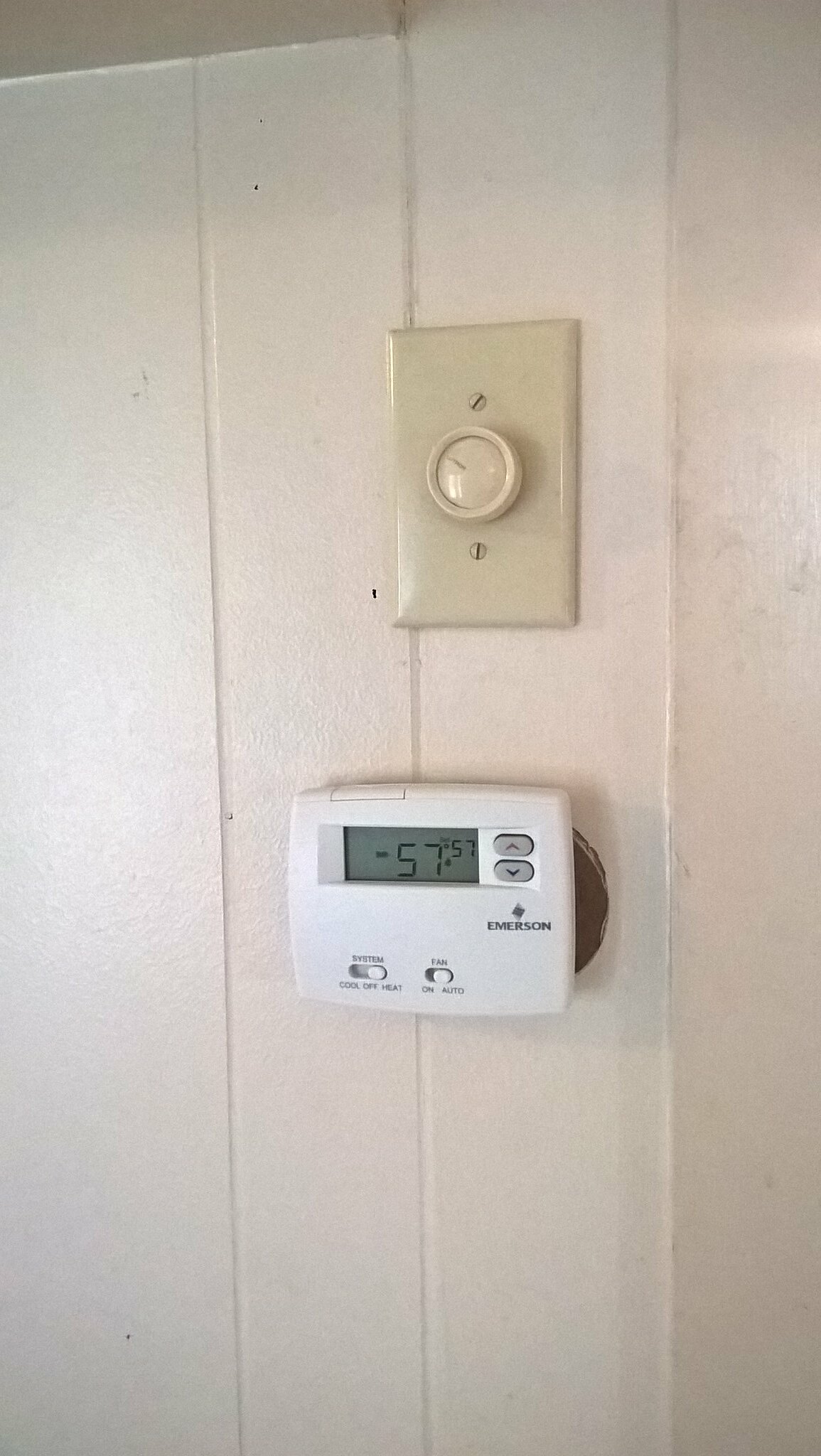This vertical color photograph captures a detailed view of a beige wall adorned with paneling lines, featuring a beige dimmer light switch and a white Emerson HVAC thermostat. The light switch, secured by two screws, has a central dial for dimming the light. Below it, the Emerson thermostat prominently displays the current temperature at 57°F and includes buttons to adjust the temperature up or down. The thermostat also features switches for selecting between cooling and heating modes, as well as for controlling the fan options—Auto, On, and Off. The detailed wall paneling complements the functional aspects of the switches, portraying a practical setup for controlling both lighting and climate within the space.